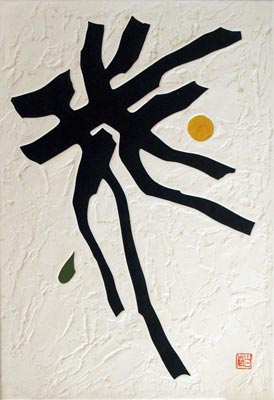The image features a striking, abstract black pattern set against a white background that resembles a textured whitewash, complete with uneven, gritty spots. The pattern, while reminiscent of Japanese or Chinese block script, is not a specific letter but rather a minimalistic, geometric design with multiple arms extending in various directions. Adjacent to the pattern, on the right side, there is an imperfect orange circle, and to the left, a green drop. In the bottom right corner, a small red square or stroke adds a final touch of color, contributing to the overall feel of a complex, intriguing abstraction.